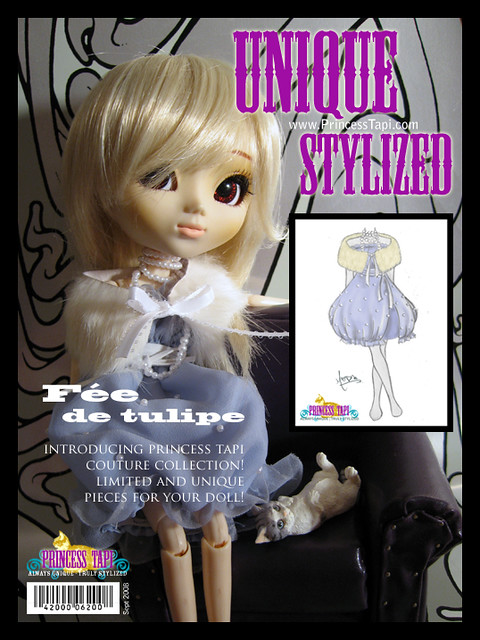The advertisement showcases the enchanting "Princess Tappi" doll from the Unique Stylized couture collection, highlighting limited and unique pieces perfect for doll enthusiasts. The doll features striking red eyes with black pupils, a fair peach complexion, and vibrant pink lips. Her long, straight blonde hair elegantly drapes over her forehead and partially covers one eye, cascading down her back.

Princess Tappi is dressed in a charming blue shirt adorned with a white faux fur wrap, complemented by a strand of white pearls around her neck. She sits gracefully on the armrest of a black leather sofa, with a small toy cat perched beside her, adding a touch of whimsy to the scene. 

Additional text in the image includes the phrases "FI DE TULIPE" and "Introducing Princess Tappi Couture Collection - Limited and unique pieces for your doll." A barcode with the number 42000006200 lies beneath the purple letters "Princess TAP," while the web address "www.princesstaupe.com" is prominently displayed in pink at the upper right corner. Adjacent to this is a black square frame containing an etching of the doll's clothing, depicting the meticulous attention to detail in her design. This magazine-style cover perfectly captures the sophisticated allure of the Princess Tappi doll and her exquisite ensemble.